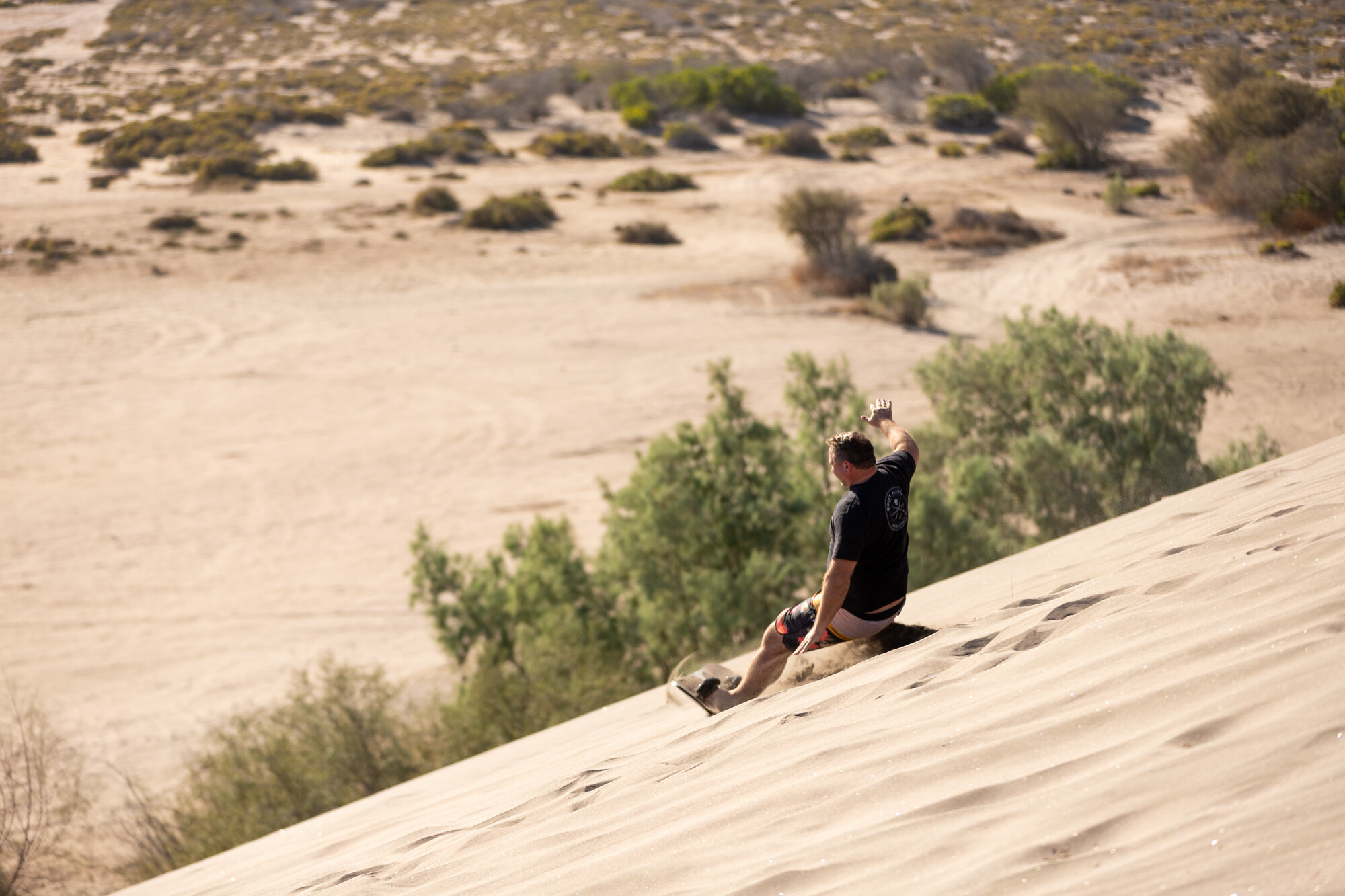The photograph captures a vibrant desert scene, characterized by dry, sandy terrain stretching into the distance. Dominating the foreground is a steep, towering sand dune. Closer to the bottom right corner of the image, a man is energetically sliding down the dune on what appears to be a sandboard, similar in shape to a snowboard. He is positioned with his legs extended forward and his buttocks barely touching the ground, possibly on a bag. He balances himself with one arm up and the other down. The man sports a black t-shirt, surf shorts, and perhaps some footwear, though it is not clearly visible. His dark hair contrasts against the golden sand. As he descends, he approaches clumps of brushy, low vegetation scattered around the base of the dune, creating a sparse yet distinct pattern of green against the expansive sandy backdrop. The distant horizon reveals more sand stretching into flat desert areas with intermittently sparse, bush-like greenery, suggesting an arid but lively environment. The overall scene evokes a sense of thrill and adventurous fun amidst the vast, striking desert landscape.